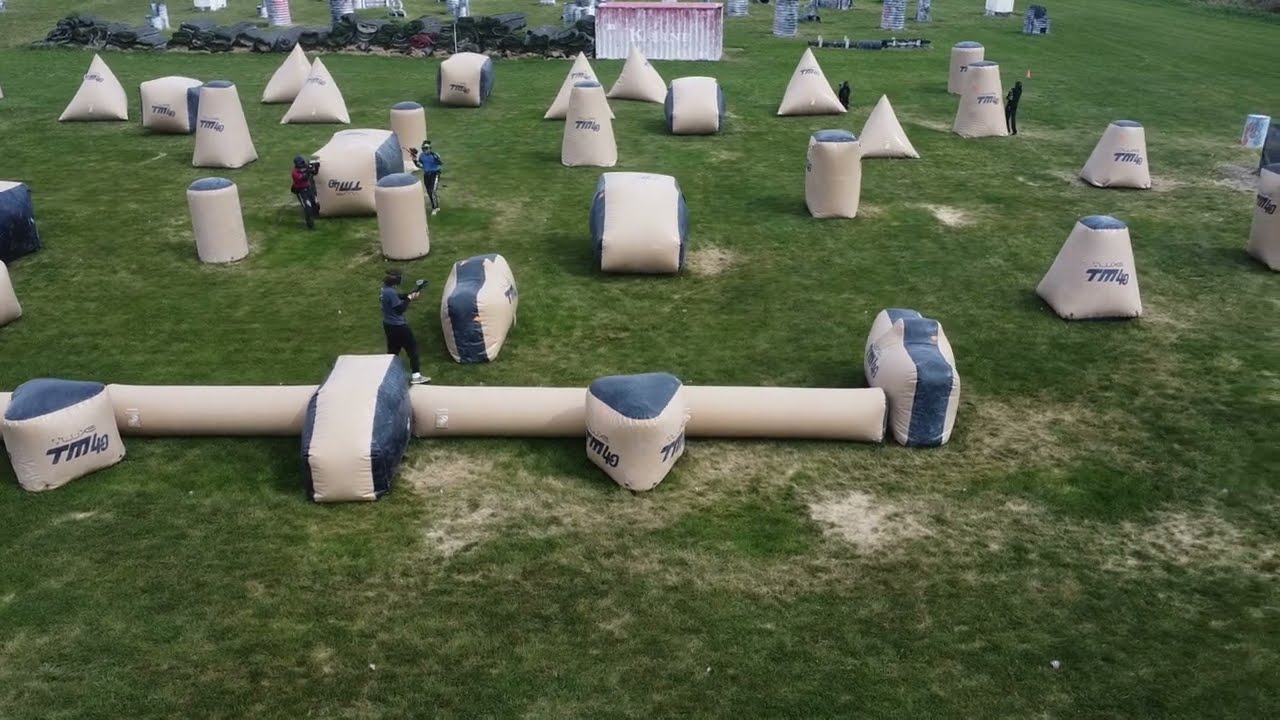The image depicts an aerial view of an active paintball field. The field is primarily grassy, interspersed with worn patches of yellowish, dry dirt, highlighting areas of frequent activity. Scattered across the field are large, inflatable obstacles of various shapes—pyramids, cylinders, and arches—marked "TM40," in beige and blue. These obstacles are designed to simulate a military environment and provide cover for the paintball players. 

There are visible gameplay dynamics, with teams donning blue and red jerseys, along with helmets. They're actively engaging, aiming paintball guns, and maneuvering behind the inflatables for cover. On the center left, a player in a red top is aiming their gun, while another in blue is raising their gun and hand in the air. Towards the top right, two players in black are positioned behind separate inflatables. 

In the background, a small shed or shipping container and another arena filled with steel barrels add depth to the setting. The image captures the strategic positioning and intense nature of the paintball match from an overview perspective.